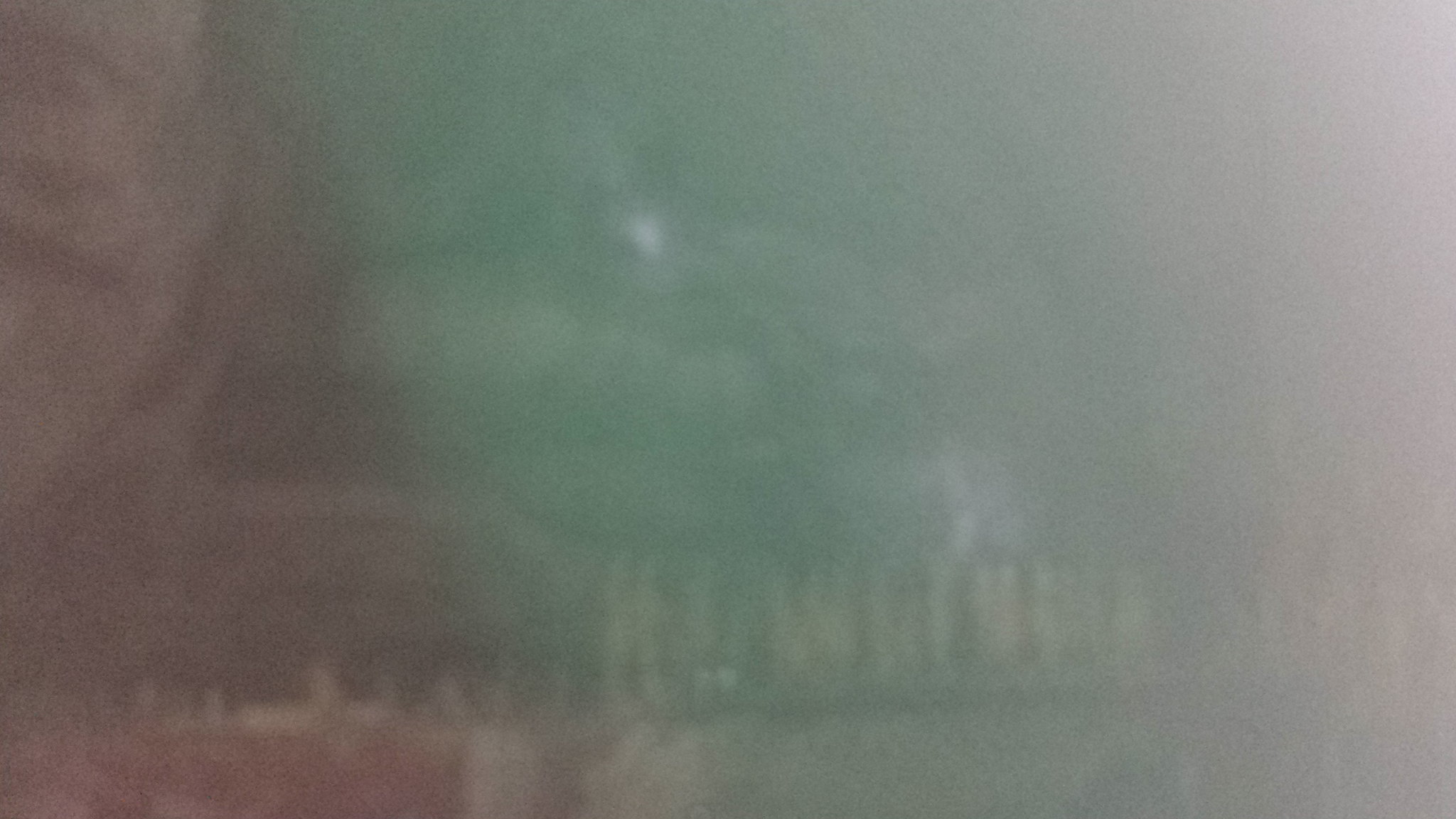In the center of this image, an abstract artwork or an extremely blurry photograph stands out. Dominating the composition, a yellow text seems to spell out a name, though only fragments of it are discernible. The name possibly begins with the letters "h-h-u-w-r-t-n-i-n-a," followed by another word starting with "s-o-f," before the text becomes indecipherable.

The image showcases a color gradient that transitions from red on the left, to green in the middle, and finally to white on the right. Adding to the mystique, the picture appears to be upside down, featuring the faint outlines of a person, with a building visible behind them. The name of the building seems to be positioned at its top, adding a layer of intrigue and complexity to the overall image.